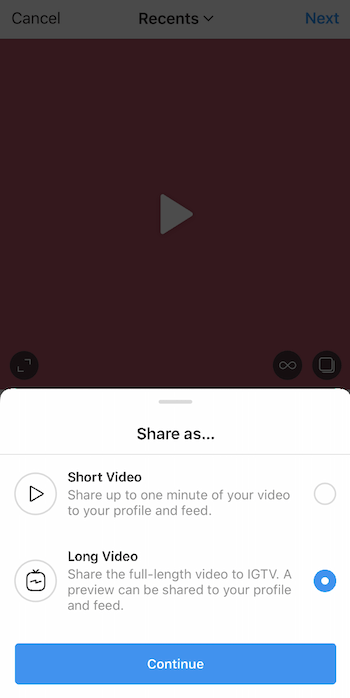The image appears to be a screenshot of a smartphone interface, possibly from a social media app, with options for sharing a video. At the very top, there is a gray-colored header with three options: "Cancel," "Recents," and "Next." In the middle of this header, there's a gray play button, though this area is somewhat blacked out, making it difficult to see clearly.

Directly below this header is a white section, under which the text "Share as..." is displayed along with an ellipsis. Below this, there's a thin gray line demarcating two sharing options.

The first sharing option is titled "Short Video," accompanied by a circular icon on its left featuring a play button. The description reads, "Share up to one minute of your video to your profile and feed." To its right is an empty circle, which indicates the option is not currently selected.

The second sharing option is titled "Long Video," and it comes with an icon resembling a TV on its left. The description states, "Share the full length video to IGTV. A preview can be shared to your profile and feed." The circle on the right of this option is filled with a blue dot, indicating it is selected.

At the bottom of the screen, there's a blue bar stretching across the width of the image, with the word "Continue" displayed in white text.